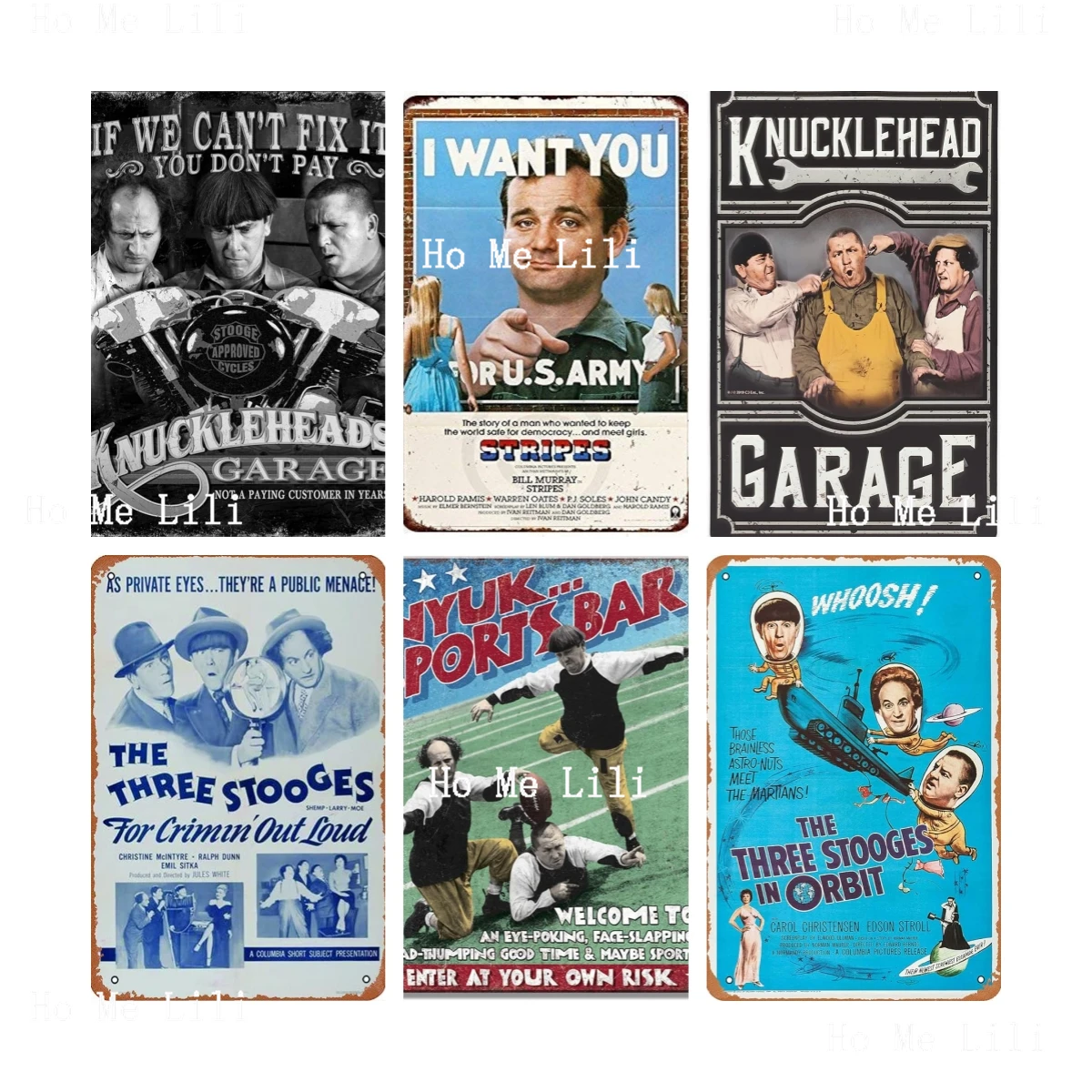This image showcases six different movie promo posters arranged in a grid of three columns and two rows. Each poster prominently features The Three Stooges, aside from the top middle one which includes Bill Murray and mimics a U.S. Army recruitment ad. The top left poster is in black and white and reads, "If we can't fix it, you don't pay—Knucklehead Garage." The top right poster is colorful and features the Three Stooges with the same Knucklehead Garage theme. The bottom left poster promotes "The Three Stooges for Crymen Out Loud" and depicts the trio set against a green backdrop in a humorous sports scene. The bottom middle one, titled "Nixxu Sports Bar," humorously shows the Stooges on a sports field, emphasizing their slapstick comedy. The bottom right poster, titled "The Three Stooges in Orbit," features an illustrated style set against a blue background, highlighting another classic theme. These vibrant, nostalgic posters, bursting with green, blue, and black hues, are perfect memorabilia for any Three Stooges fan.